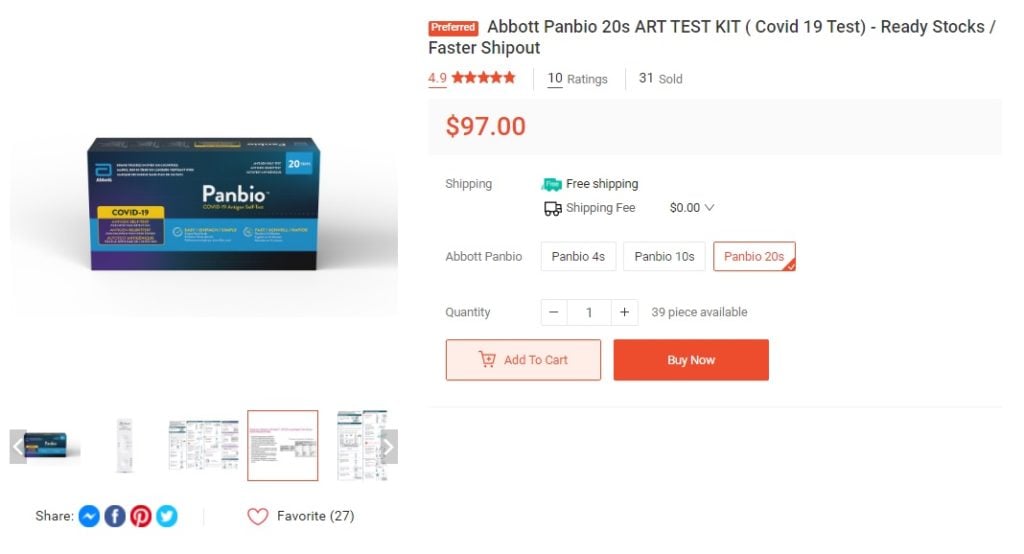The image resembles a printout of a web page featuring the Abbott PanBio COVID-19 testing kit, specifically the 20-pack version. Dominating the left side is a high-resolution photograph of the PanBio kit’s packaging, characterized by vivid colors on a blue background with a prominent yellow COVID-19 emblem. The product title and highlights are displayed in vibrant orange text, denoting it as the "Abbott PanBio 20s Art Test Kit (COVID-19 Test)," emphasizing its ready stock and fast shipping options.

The product has garnered impressive user feedback, evidenced by a rating of 4.9 out of 5 stars based on 10 reviews, with 31 units sold. Priced at $97, the kit is available with free shipping. The page allows for selection among various packaging options, including PanBio 4s, 10s, and 20s; in this instance, the 20s pack is chosen, with a single unit selected from the 39 available. 

An orange "Buy Now" button, accompanied by a shopping cart icon and "Add to Cart" option, is prominently featured, suggesting an active selection. Below the main section are clickable monochromatic thumbnails likely leading to additional product information. Social media sharing options including Twitter, Facebook, and more are positioned nearby, alongside a "Favorites" button indicating that 27 users have favorited this item.